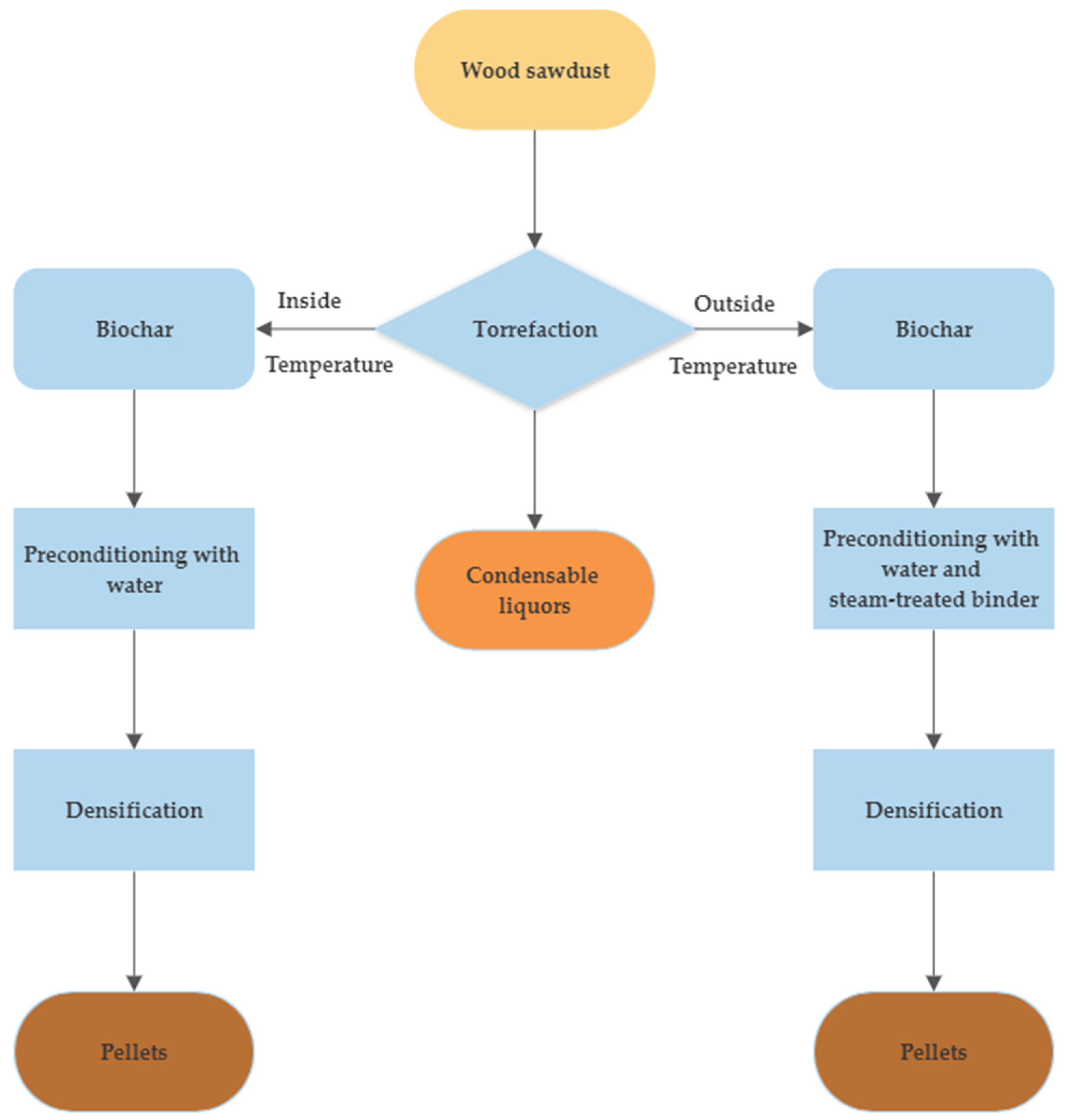The image features a detailed diagram on an all-white background with multiple shapes and arrows denoting a process. At the top center is a yellow, rectangular oval labeled "Wood Sawdust" in black text. A dark blue arrow points downward to a central blue diamond that reads "Torrefaction." From this diamond, two sets of arrows extend. 

On the left, a dark blue arrow labeled "Inside Temperature" points to a light blue rectangular box labeled "Biochar." Another dark blue arrow points downward to a blue rectangle labeled "Preconditioning with Water." Below this, a dark blue arrow leads to another blue rectangle reading "Desiccation." A final dark blue arrow descends to a dark orange, rectangular oval reading "Pellets."

To the right of the central diamond, another dark blue arrow labeled "Outside Temperature" points to a light blue rectangular box also labeled "Biochar." From here, a dark blue arrow points downward to a blue rectangle labeled "Preconditioning with Water and Steam Treated Binder." Another dark blue arrow points down to a blue rectangle labeled "Densification," followed by a final dark blue arrow pointing to a dark orange, rectangular oval marked "Pellets."

Additionally, directly below "Torrefaction," another blue arrow points downward to a dark orange, rectangular oval labeled "Condensable Liquors." The diagram is organized in a manner reminiscent of a flowchart or mind map, detailing a specific process with emphasis on color-coded shapes and directional arrows facilitating the progression of information.